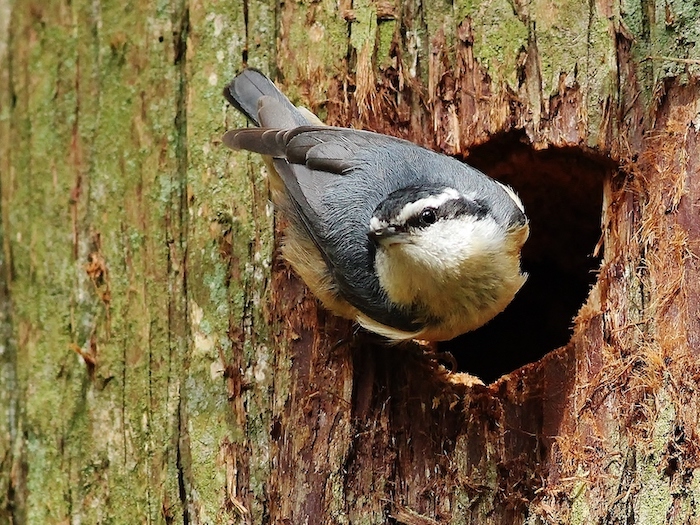The photograph captures a surprising moment in nature. A small, yellow and black bird with a distinctive white or tan neck peers out from a dark, hollow hole within a large, ancient tree trunk. The trunk, textured with rich wood grain, displays a captivating mix of brown hues on its right side, seamlessly blending into a vibrant green moss that dominates the left side and parts of the top and bottom right corners. The bird is perched delicately on the bottom edge of the hole, its startled expression suggesting it might have just been disturbed. The image, potentially taken with a phone or camera as part of nature photography, focuses sharply on the bird and the intriguing interplay of colors and textures of the moss-covered tree, providing a vivid glimpse into the natural world without any accompanying text.